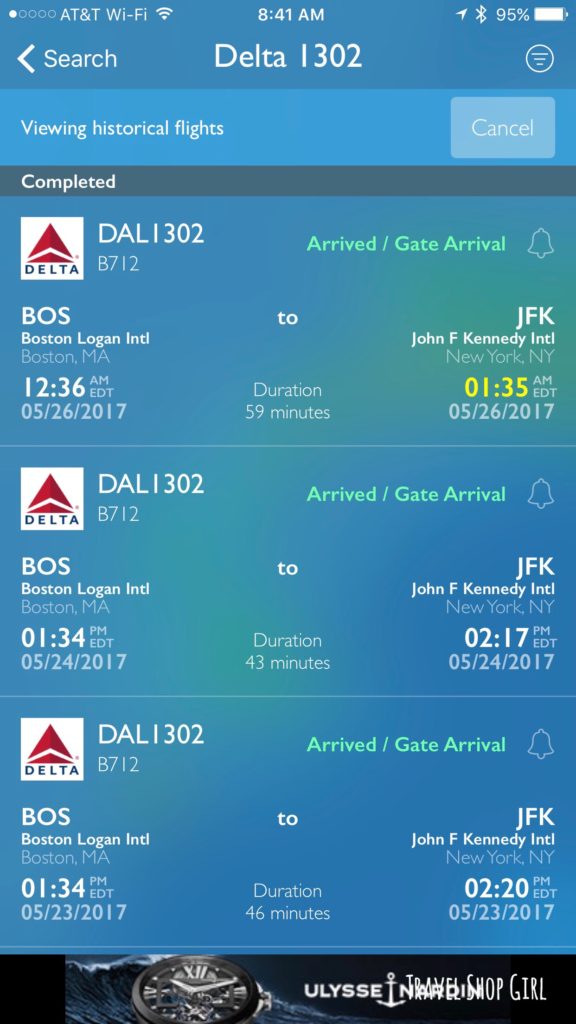The image captures a screenshot of someone's cell phone display showcasing a flight itinerary with Delta Airlines. The background is predominantly a tranquil, sky-like blue, reminiscent of a clear day. In the middle, there's a subtly hazy green area that adds a touch of depth to the backdrop. At the top of the screen, the text indicates it’s a search result for "Delta 1302" under "Viewing Historic Flights." The status of the flight is marked as "Completed."

The itinerary details a flight from Boston to John F. Kennedy International Airport (JFK) with a gate arrival time of 1:35 PM. The trip spanned from May 23, 2017, to May 26, 2017, and included stops or events each day. Delta's emblem, featuring a white square with red triangles, is prominently displayed at the top, adding brand recognition and coherence to the document's layout. The image is rich with flight details, including various dates, times, and locations, providing a comprehensive overview of the traveler's journey.